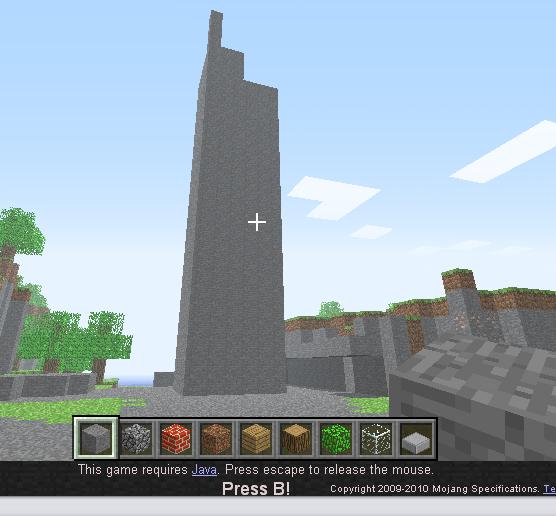This image is a detailed screenshot from the popular sandbox game, Minecraft. Dominated by the game's signature cube and rectangular shapes, the scene centers around a player constructing a towering monolith-like structure using gray stone bricks. The builder’s inventory is visibly displayed at the bottom of the image, showcasing a variety of items such as stone, brick, wood, leaves, and glass, indicating a diverse collection of materials.

The backdrop portrays a clear, sunny day within the Minecraft world, characterized by a vibrant blue sky and scattered white clouds. To the left of the structure, a cluster of trees enhances the natural landscape. On the right side of the image, evidence of excavation is apparent where the player has mined into the mountainside, likely gathering the necessary resources for their construction project. The scene epitomizes a typical day of creative and resourceful building in the vast, blocky universe of Minecraft.